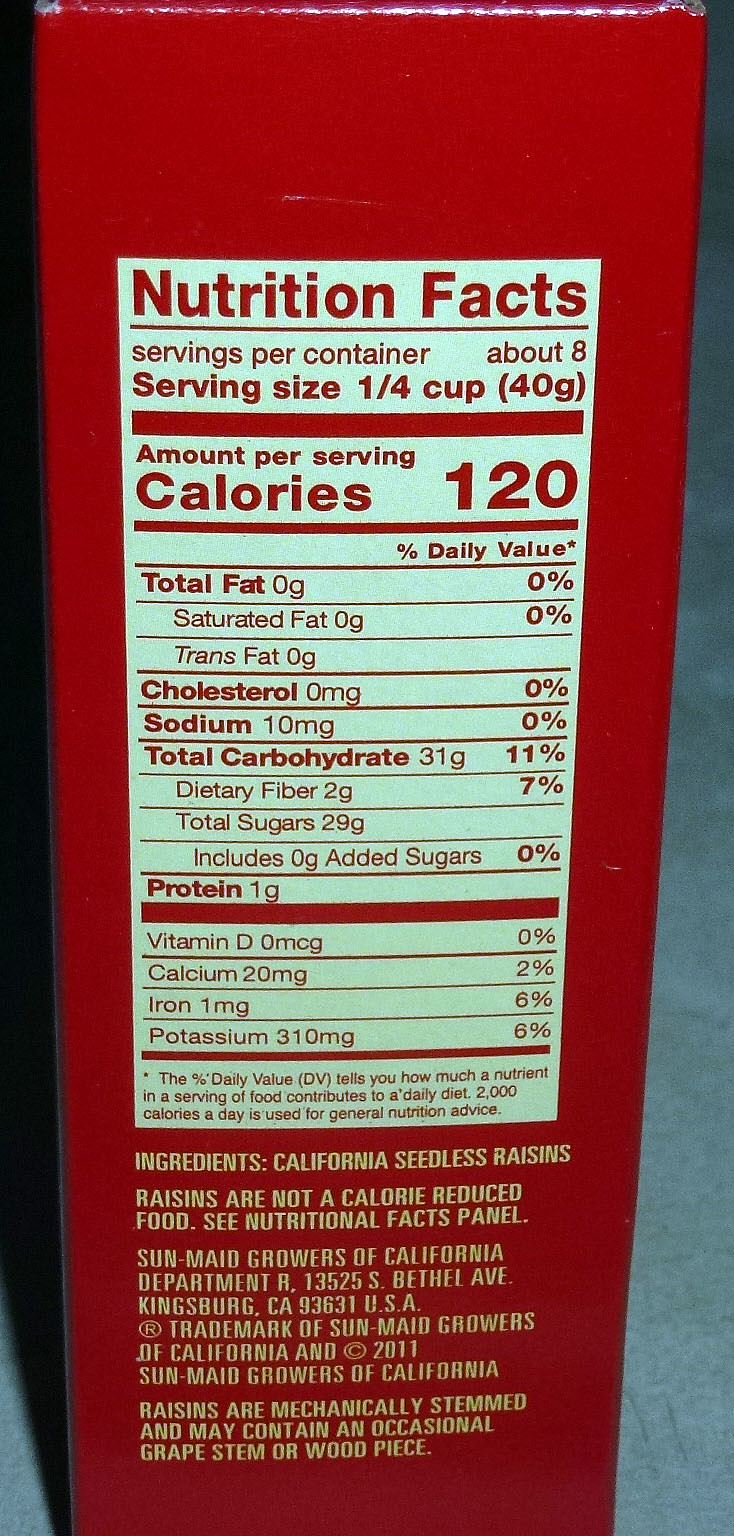This image features a tall and narrow photograph showcasing the side of a red box of Sun-Maid raisins. The primary focus is the nutrition facts label, which stands out prominently against an off-white background. The label details that the product contains approximately eight servings per container, with each serving size being a quarter cup or 40 grams, amounting to 120 calories per serving. Below the calorie count, the label lists the daily nutritional values.

At the bottom of the nutrition label, the sole ingredient listed is "California seedless raisins." Additionally, there is a disclaimer that reads, "Raisins are not a calorie reduced food. See nutrition facts panel." The label also notes that the raisins are mechanically stemmed and might occasionally contain grape stems or small pieces of wood. The packaging further identifies the manufacturer as Sun-Maid Growers of California, along with their address.

The caption encapsulates the comprehensive details and disclaimers presented on this classic red box of Sun-Maid raisins.